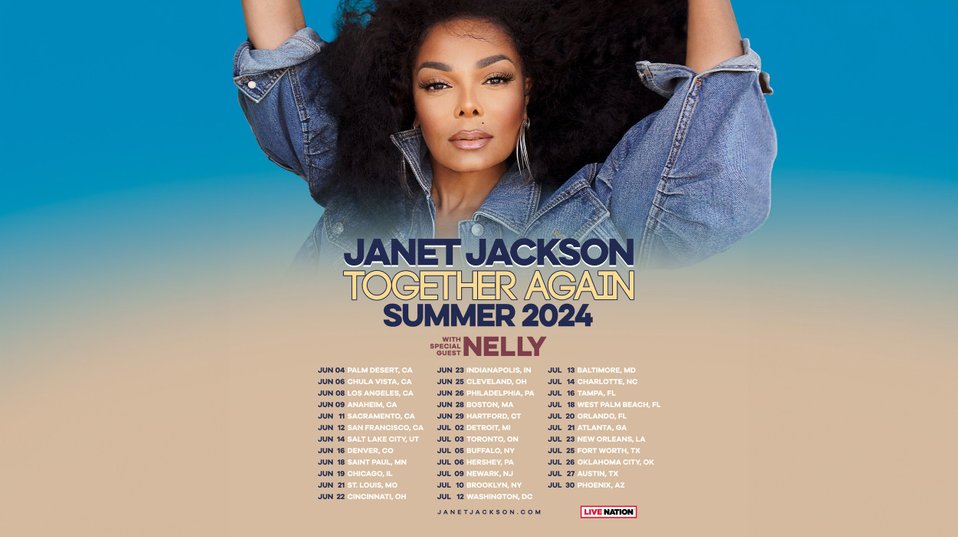The poster for Janet Jackson's "Together Again" Summer 2024 tour, brought to you by Live Nation, features Janet centered prominently against a vivid blue and nude-colored gradient background. Janet Jackson's dynamic pose showcases her raised arms extending out of the frame, emphasizing her energetic stage presence. She is dressed in a denim shirt with sleeves rolled down to her elbows, adorned with large round silver hoop earrings and wearing defined makeup with lipstick. Her hair is voluminous and natural, adding to her iconic look. The poster includes text details: Janet Jackson's name in blue, "Together Again" in yellow, "Summer 2024" in blue, and "With Special Guest Nelly" in red. Below, it lists the concert dates, cities, and venues in blue and white lettering. A website, JanetJackson.com, is provided for more information. All elements are centrally aligned, guiding the viewer's focus from Janet Jackson to the tour information seamlessly.